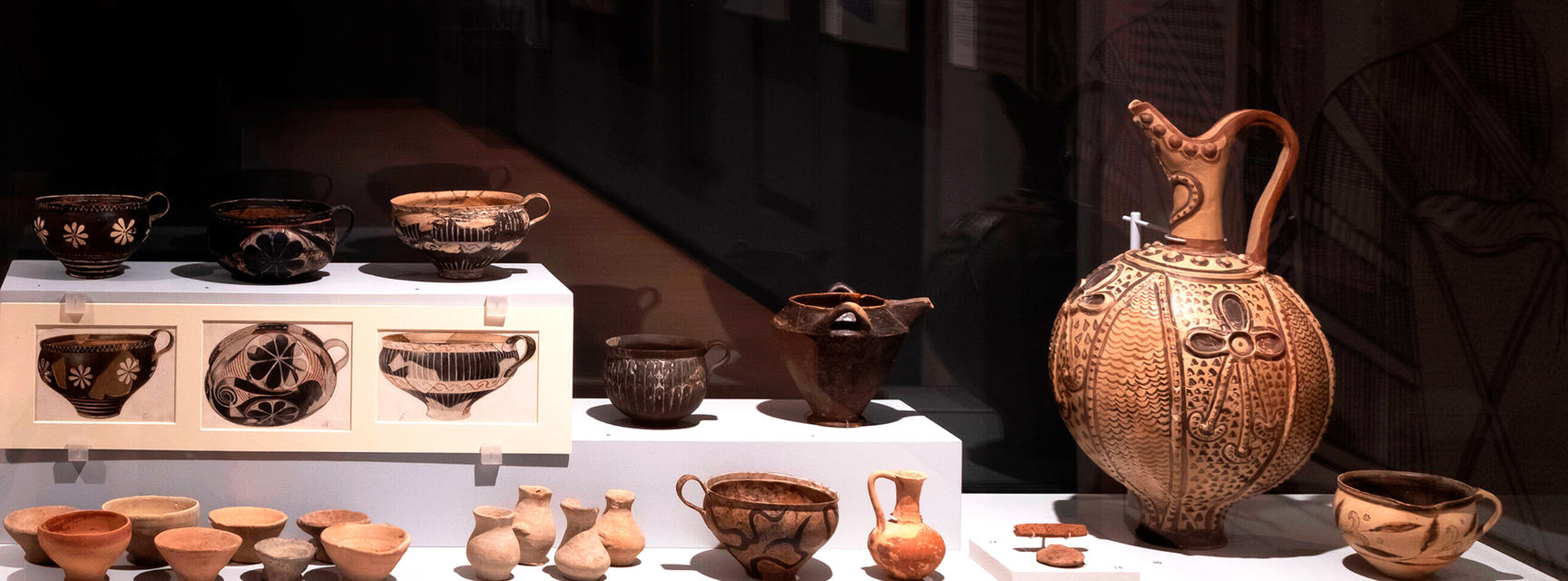The photo captures an exhibit of ancient pottery displayed on white pedestals in a museum setting. The centerpiece is a large, bulbous urn with intricate carvings, including a floral design and a rope pattern encircling its light brown surface. This striking urn narrows elegantly at the neck, adding to its decorative appeal. Surrounding it are various pieces, including simple earthenware cups made from plain clay, small vases, and bowls. Notably, there is a small brown teapot and some cups with handles that are painted and more ornate compared to the predominantly natural clay items. On the lower tier of the display, there is another jug, numerous small cups and bowls, and four additional small vases. To the right, a giant jug adorned with detailed drawings stands prominently. The exhibit is accompanied by a diagram providing information about the pieces, enhancing the educational value of the display. The background is dark, which contrasts with the light cloth on the table, further highlighting the pottery's historical and artistic significance.